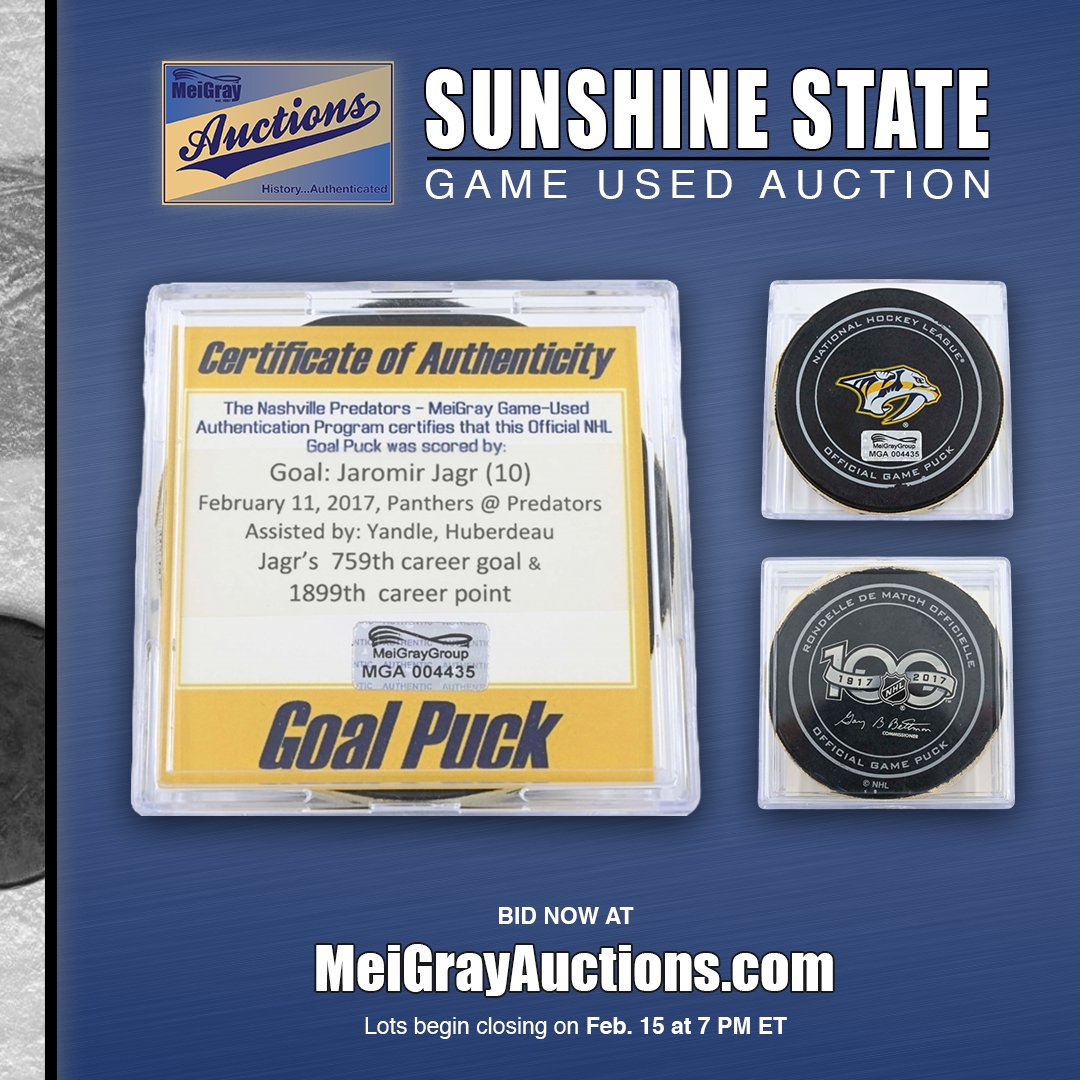This image is an advertisement for an auction hosted by MEI Gray Auctions, showcased on a blue background. At the top left, it reads "MEI Gray Auctions" with "Auctions" in blue cursive font and a fancy swirling triangle underneath. The headline, "Sunshine State Game Used Auction," is displayed prominently with "Sunshine State" in bold white font and "Game Used Auction" in capitalized white font. Below this, the phrase "History Authenticated" leads into a detailed Certificate of Authenticity.

The certificate states that the Nashville Predators-MEI Gray Game-Used Authentication Program certifies the authenticity of the official NHL goal puck. Specific details include that the goal puck was scored by Jeremy Jag10 on February 11, 2017, during a game between the Florida Panthers and the Nashville Predators. The goal was assisted by Yandel and Hoover Day, marking Jagger's 759th career goal and 1,899th career point. The certification is labeled with the identifier MGA-004435.

To the right of this informative board, the image displays two goal pucks showcasing the official NHL logo, a jaguar head emblem, and the inscription "100" to commemorate 100 years, with the year 2017 prominently featured. The distinctive design of the pucks underscores their authenticity.

At the bottom of the advertisement, it urges viewers to "Bid now at meigrayauctions.com," noting that the lots will begin closing on February 15th at 7 p.m. ET.